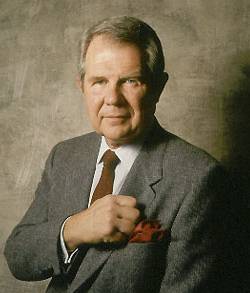In the photograph, a middle-aged Caucasian male with short, grayish-brown hair and light-colored eyes is wearing a dark gray suit, a white button-up collared shirt, and a red tie. A red handkerchief is neatly tucked into the breast pocket on the left side of his suit. His right arm is bent at the elbow, with his right hand making a fist over his heart. The man is facing the camera with his body slightly turned to the left, displaying a semi-smile on his jowly face. The background is a textured grayish-brown, featuring areas of shadow, particularly in the middle and lower right, giving the scene a nuanced lighting effect.